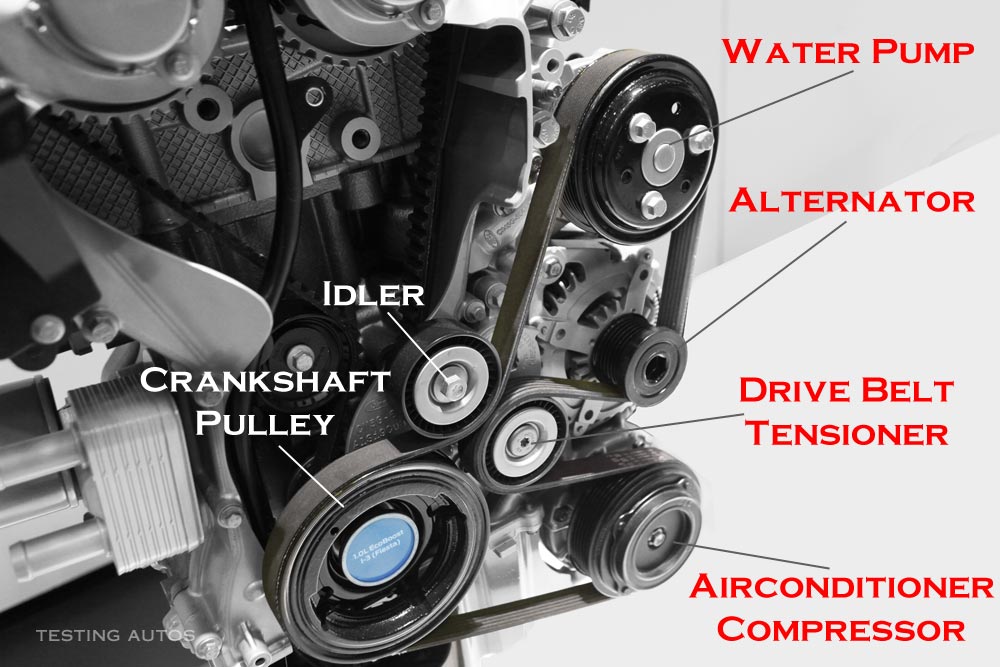The image is a detailed diagram of the internal components of an engine, primarily focusing on the drive belt and its associated parts. The engine occupies about two-thirds of the picture and is rendered in gray or silver tones. The diagram uses red font to label components on the right and white font for those on the left. Starting from the top right and moving downward, the labeled parts include the Water Pump at the top, the Alternator below it, the Drive Belt Tensioner in the middle, and the Air Conditioner Compressor at the bottom right. On the left side, the Crankshaft Pulley is identified in white font near a small blue circle, with the Idler positioned above it. All these circular components, resembling pulleys, are connected by a black rubber drive belt. Additional text in the lower left corner of the image reads "Testing Autos," suggesting that this diagram might be intended for instructional or diagnostic purposes in an auto shop. The overall image provides a clear and organized depiction of how the drive belt interconnects various engine parts.